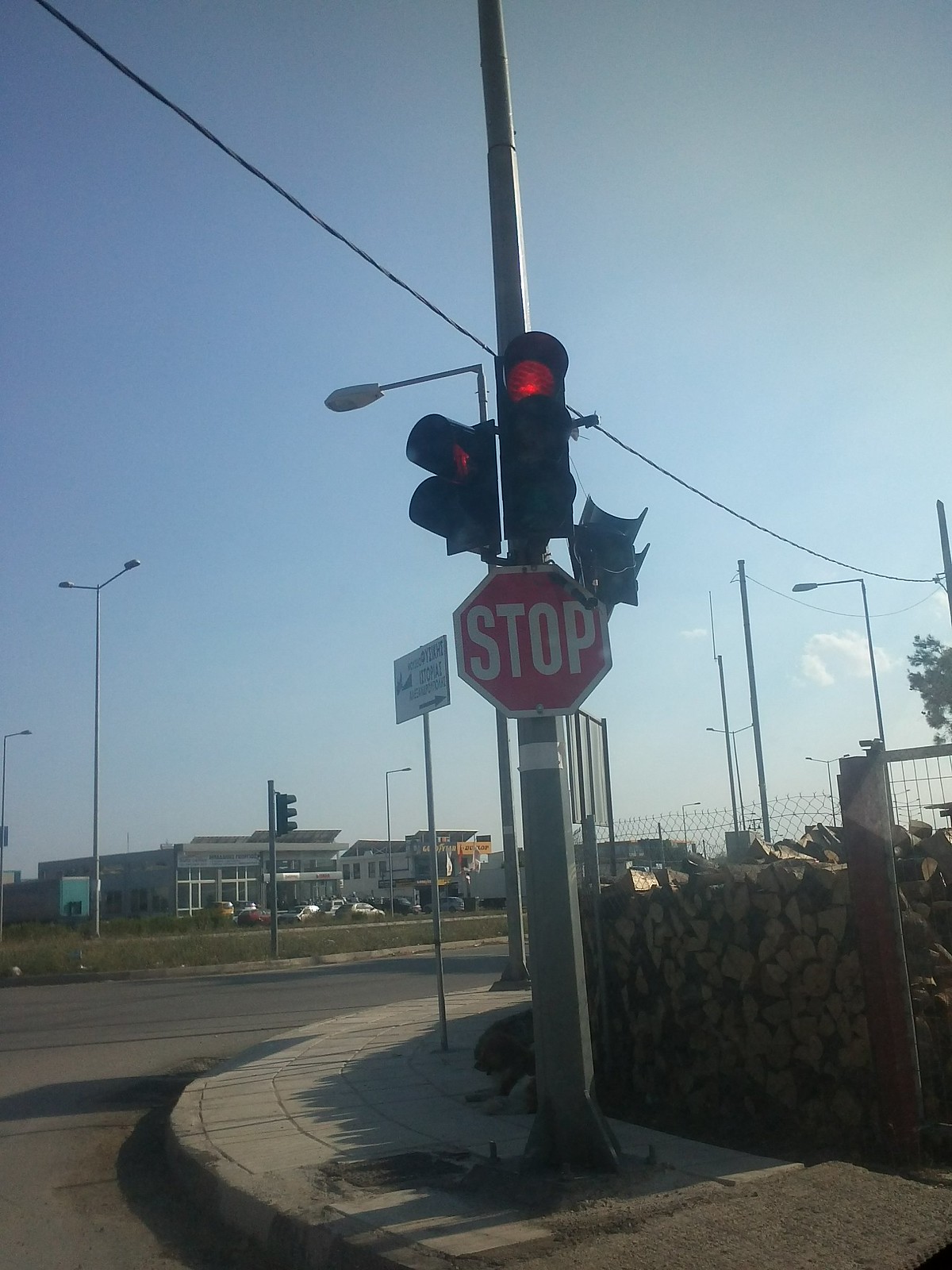The photograph captures an urban intersection under a clear blue sky, featuring a prominent stoplight and stop sign mounted on a large gray metal pole on a paved city sidewalk. The stop sign, a standard red octagon with white reflective text reading "STOP," is positioned below the dual stoplights. One stoplight has two lights, including a red one, while the other has three, also displaying a red light. The background reveals a fenced yard to the right with piles of firewood, indicating a possible lumber business. To the left and further back, multiple buildings are visible, including what appears to be a glass-fronted warehouse or car dealership with several cars parked in front. Additional streetlights and various poles extend over the street, while sparse shrubbery can be seen directly behind the traffic light pole. The scene suggests a bustling four-way intersection, encapsulated by the surrounding businesses and residential structures.